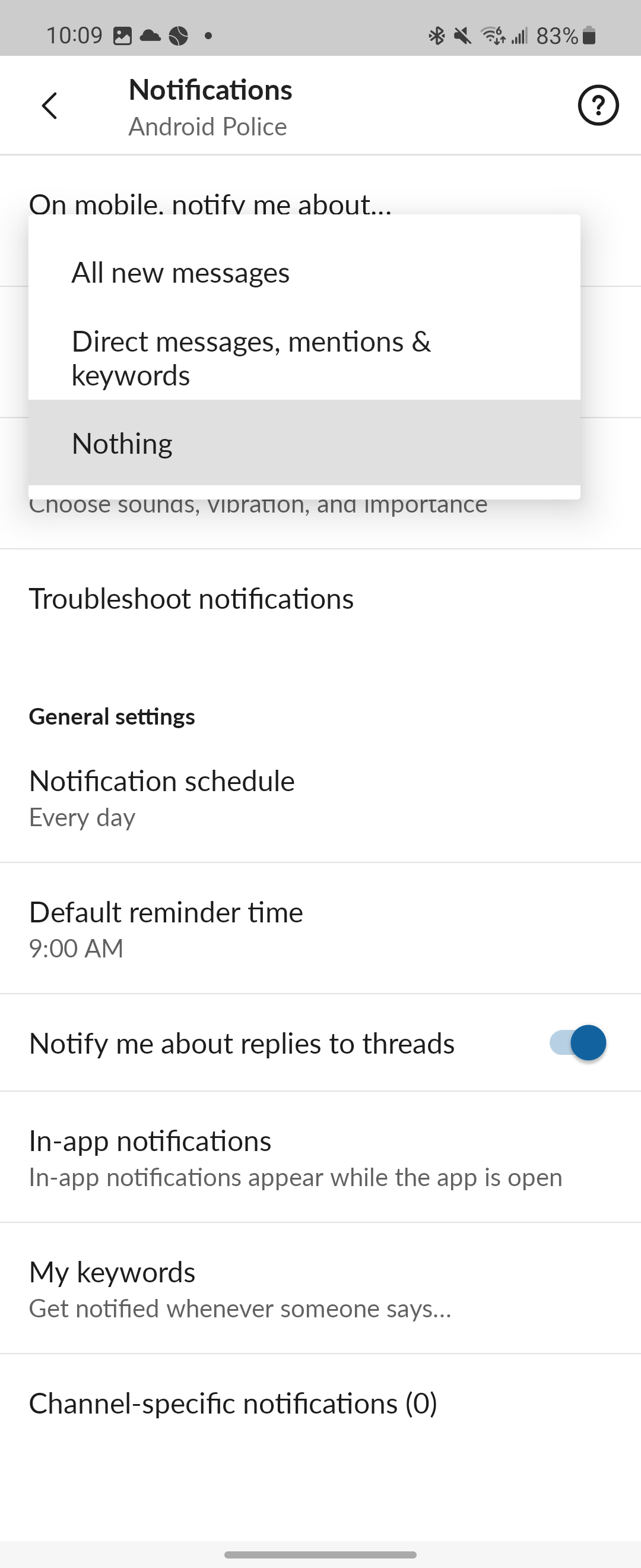A detailed screenshot of a phone notification settings page appears. 

At the top, a gray and black status bar displays essential information about the device, such as battery level, Wi-Fi connectivity, Bluetooth status, and the current time. 

Directly below the status bar is a white section with black text reading "Notification Android Police." An arrow points to the left, and a question mark enclosed in a black-lined circle is present as a help icon.

The main content area begins with the header "On Mobile, Notify Me About," followed by a pop-up window with multiple notification options: "All messages," "All new messages," "Direct messages," "Mentioned keywords," with none of them selected.

Further details include options to "Choose Sounds, Vibration, or Importance” for notifications. 

The page also highlights several settings options such as "General settings," "Notification settings," "Everyday settings," "Default time reminder," and an active "Notify Me" toggle.

Below are settings pertaining to "In-app notifications," "My keywords," notifications when "Someone" is specified, and "Channel-specific notifications."

At the bottom of the screenshot is a small, tiny gray box with a dark gray horizontal line, likely indicating the draggable area for the pop-up window.